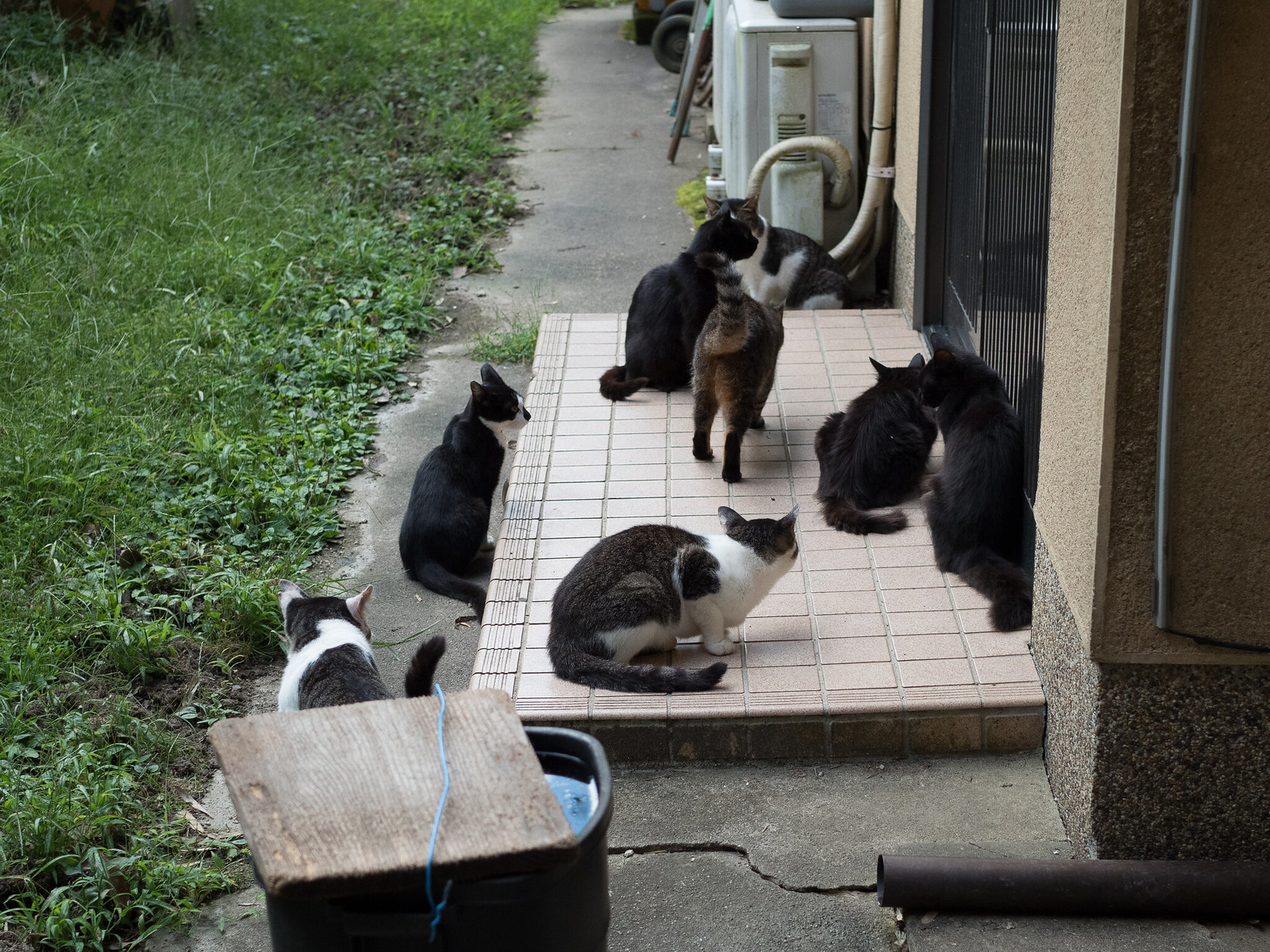In this color photograph, eight cats—mostly black or black with white patches—are lounging on a small, elevated, checkered patio situated just outside a building's sliding door. The greyish building features descending pipes and what appears to be an air conditioning unit above the cats. To the left of the image is a grassy yard transitioning into the grey slab patio, which is bordered by a paved path. A brown wooden cube with a blue thread and a round object containing blue liquid are also visible in the foreground. This image, captured in daylight, showcases the mixed textures and colors of the environment and highlights the plethora of feline inhabitants, with one or two displaying a brownish hue.